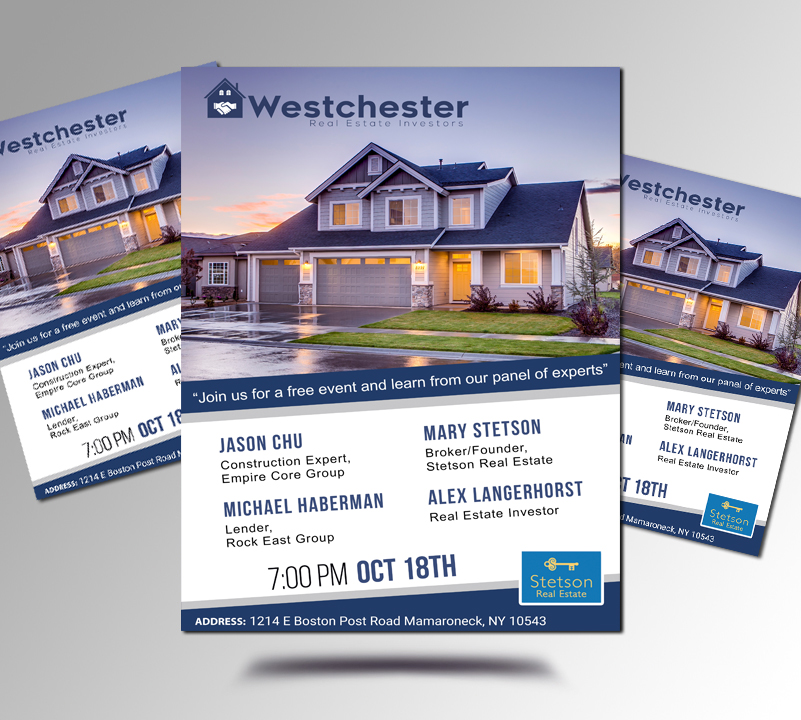The image showcases an advertisement flyer for Westchester Real Estate Investors, prominently displayed three times in an overlapping manner with a grey background. The central poster, the focus of the display, features a vibrant photograph of a multi-bedroom house with a manicured lawn, driveway, and surrounding neighborhood. At the top of the poster in blue text, it reads "Westchester Real Estate Investors," accompanied by a logo of a blue house with white handshake graphics in the top left corner. Below the photograph, a heading invites viewers to "Join us for a free event and learn from our panel of experts." Further down, the flyer lists the names of the panelists and their titles in blue text: Jason Chu, Construction Expert from Empire Core Group; Mary Stetson, Broker-Founder of Stetson Real Estate; Michael Haberman, Lender from Rock East Group; and Alex Langerhorst, Real Estate Investor. The event is scheduled for 7 PM on October 18th at Stetson Real Estate, located at 1214 East Boston Post Road, Mamaroneck, New York, 10543. The bottom right corner features the Stetson Real Estate logo, marked by a blue background, white font, and a white key symbol. The two side posters replicate this central design but are slightly tilted and partially hidden behind the main poster.